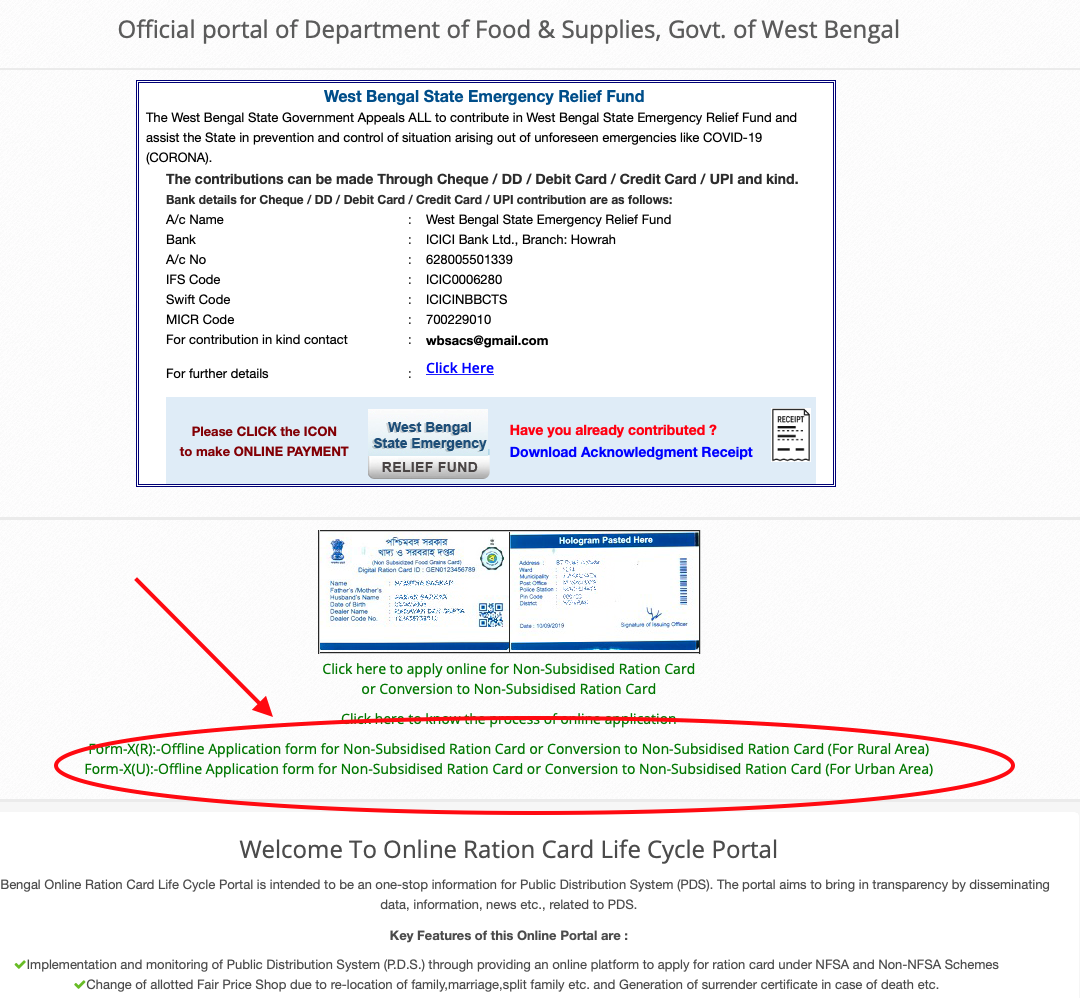**Descriptive Caption:**

The image captures a webpage titled "Official Portal of the Department of Food and Supplies, Government of West Bengal." Dominating the upper section, a box highlights the "West Bengal State Emergency Relief Fund." This box details an appeal from the West Bengal state government, urging citizens to contribute to the fund to aid in the prevention and control of emergencies, exemplified by the COVID-19 pandemic. Contributions can be made through various channels including cheque, demand draft (DD), debit card, credit card, UPI, and in-kind donations. The box provides specific bank details for these contributions and concludes with a prompt: "For further details click here." At the very bottom, another prompt urges users to "click the icon to make an online payment" via a button labeled "West Bengal State Emergency Relief Fund."

On the right side of the box is a query, "Have you already contributed?" followed by an option to "Download Acknowledgement Receipt."

Below this section are two side-by-side images that contain extensive text, though the details within these images are unclear. Beneath these images is a call-to-action: "Click here to apply online for a non-subsidized ration card or conversion to a non-subsidized ration card."

Highlighted further is a red circle with an arrow directing attention to a form titled "Offline Application Form for Non-Subsidized Ration Card or Conversion to Non-Subsidized Ration Card." This form is split into two sections based on residential areas, with the top part labeled "For Rural Area" and the bottom "For Urban Area".

Finally, another section welcomes users to the "Online Ration Card Lifecycle Portal," accompanied by additional small text that provides further details.